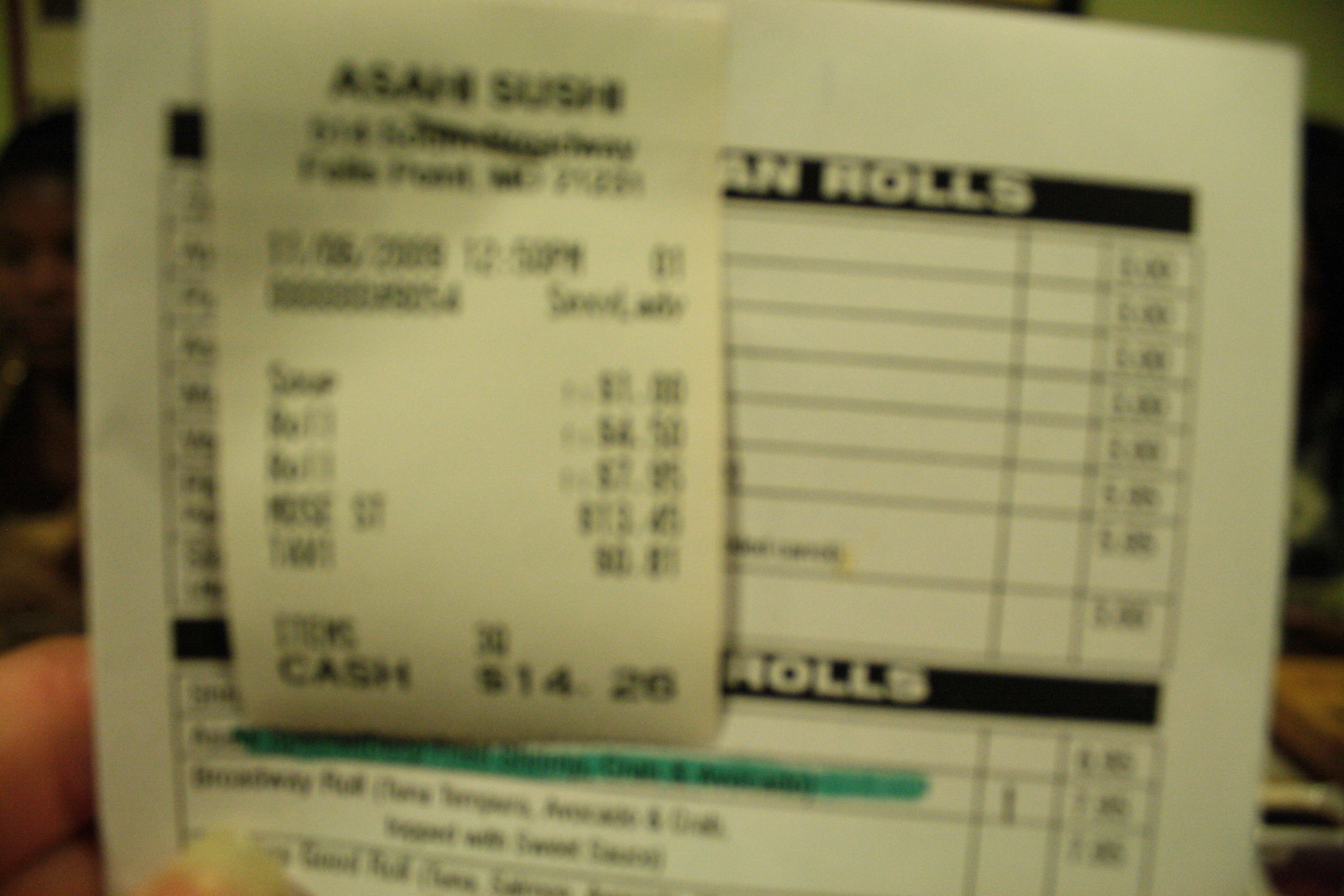A faded and blurred receipt, taped to a sheet of paper detailing roll prices, occupies the center of the image. The store name is illegible, but the transaction amount is visible at $14.20. Highlighted in blue is the price of the second roll listed in the second section, possibly indicating the purchased item or an issue of note. A woman, identifiable by her long nails, is holding the paper, with just her hand and fingers visible against a gray background.